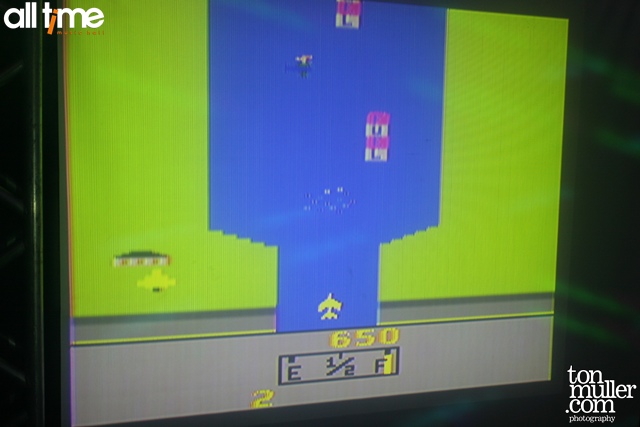The color image is a rectangular, horizontal photograph of an old, vintage, pixelated computer game screen, evocative of 1980s arcade games. This photograph was taken from a slight angle to the left, making the right side appear farther away. At the bottom right corner, the copyright or ad reads "tonmuller.com photography" in lowercase white letters on a black background. 

In the game screen's upper left corner, "all time" is written in lowercase Arial letters, with the 'i' in orange and slanted. Below it, there's an illegible orange text. The background of the screen is bright green with a prominent blue strip or runway/bridge running down the middle. At the bottom middle of this blue strip is a small yellow airplane or fighter jet that the player likely controls. Another identical jet is located farther to the left on the yellow background, adjacent to the runway/bridge.

Below the blue strip, along the bottom of the screen, there is a gray background occupying about two-fifths of the screen. On this gray background, directly under the aircraft, the number "650" is written in yellow. Below this number is a fuel gauge represented by a white rectangle with three notches, labeled 'E' on the left, '1/2' in the middle, and showing the fuel tank approximately three-quarters full. A small pixelated house is also depicted in the lower left corner of the screen, reinforcing the nostalgic, retro gaming aesthetic.